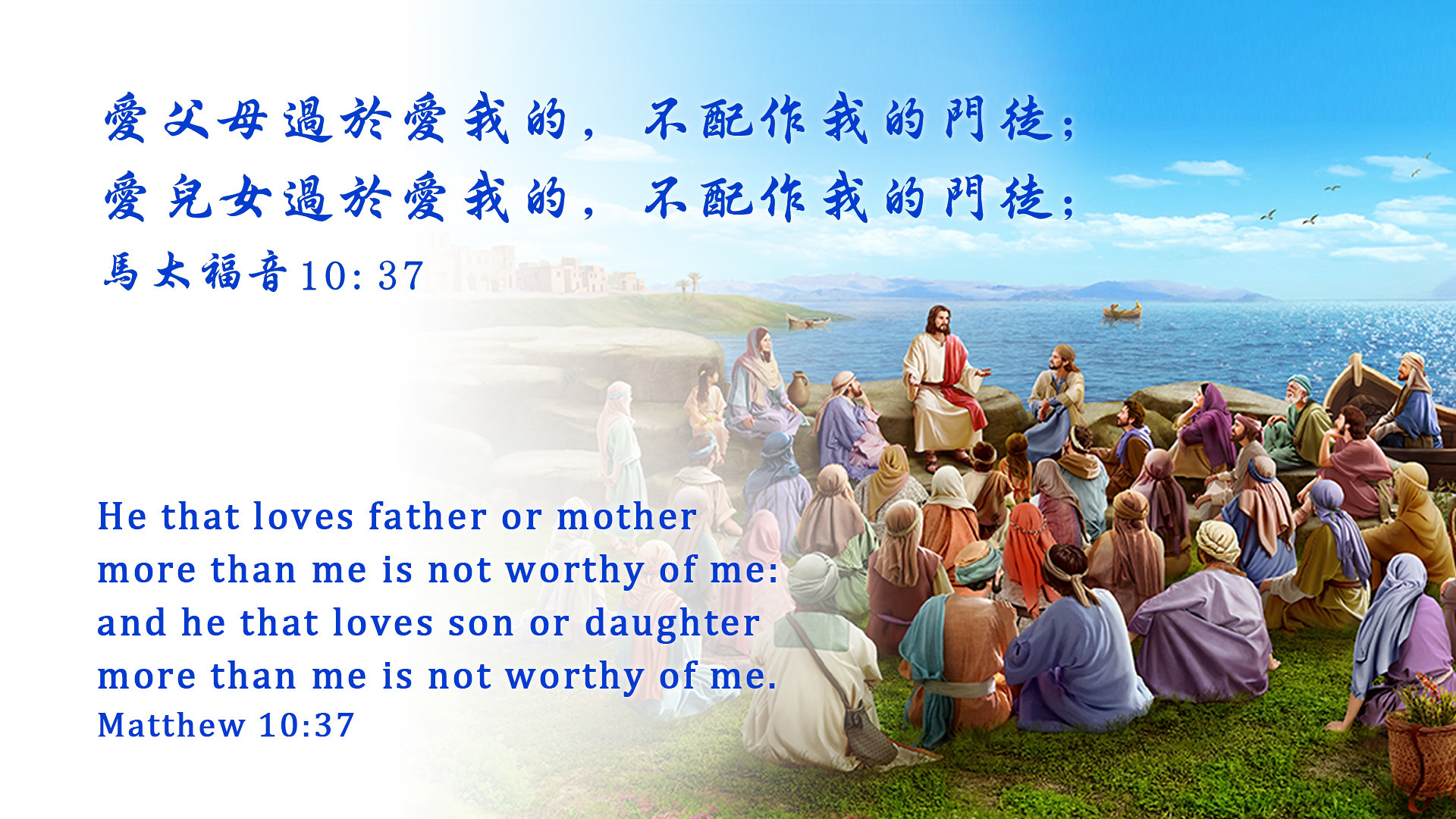The artistic piece is a vibrant and detailed painting depicting Jesus Christ surrounded by a crowd of people. Jesus is seated on a rock ledge overlooking a serene body of water, with a brown boat visible on the blue waters, and a city and mountains can be seen in the distant background. The gathering includes men, women, and children, all wearing colorful attire typical of the era, with gowns in shades of purple, blue, tan, and white, and various hats. Some of the people sit on green grass, while others are perched on gray or tan rocks, and a person in a blue gown is seated in the boat. Behind some of the people, a brown basket filled with green foliage is visible. The sky transitions from white on the left side to blue on the right. At the top of the artwork, a prominent blue text written in Chinese spans across half the page, while at the bottom left, the English translation reads: "He that loves father or mother more than me is not worthy of me. And he that loves son or daughter more than me is not worthy of me. Matthew 10:37." Both messages emphasize the importance of devotion to Jesus above familial bonds.